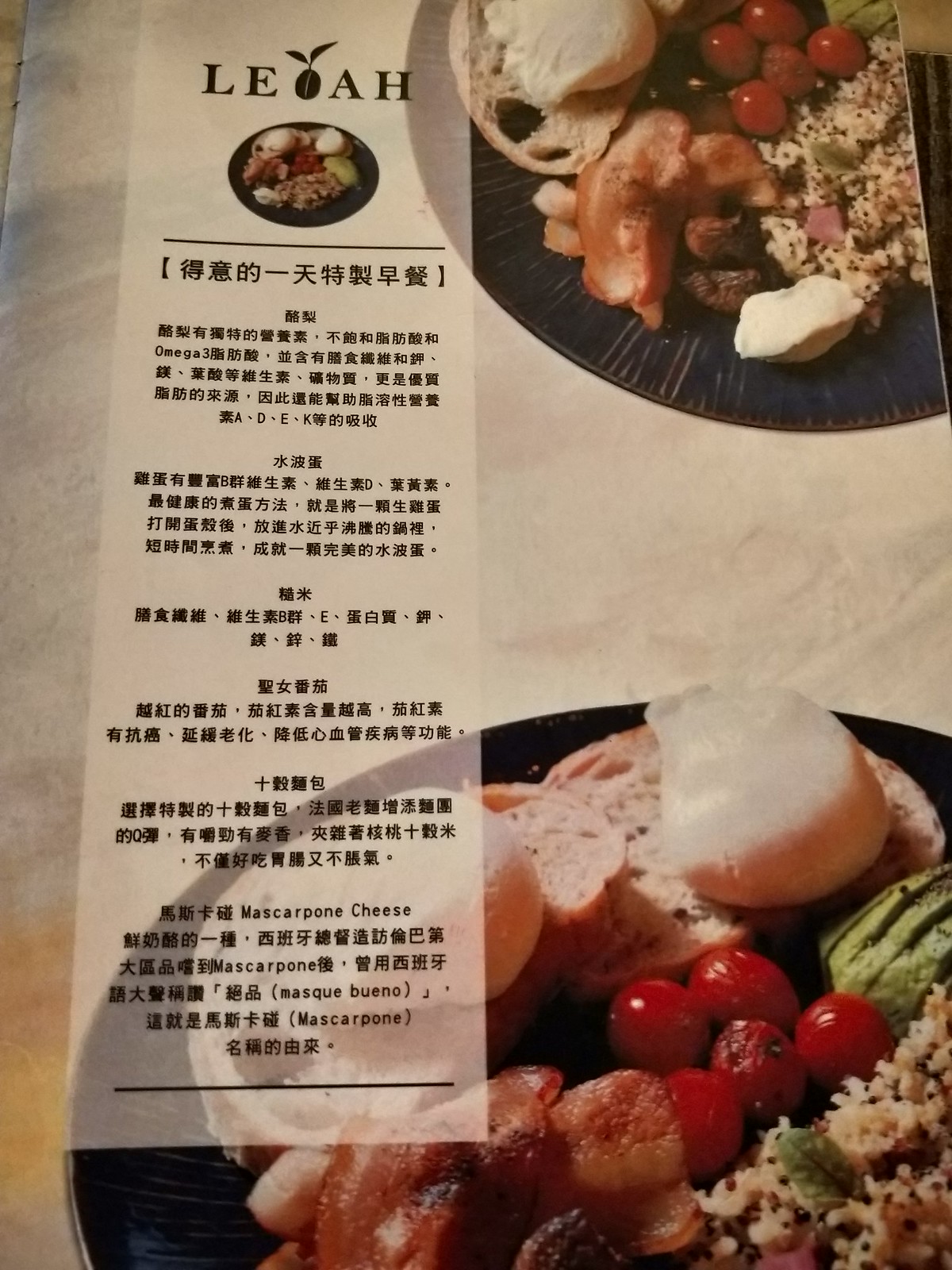The photograph showcases a menu predominantly in Japanese characters. Prominently featured in English is the name "Leah," in segmented letters "L-E," followed by an image of what appears to be a plum, and then "A-H," spelling out "Leah." The menu includes two inset images of food dishes: one displaying a slice of bread topped with a creamy spread, cherry tomatoes, and the other showcasing a rice dish garnished with a green leaf, possibly for seasoning. Towards the bottom section of the menu, likely the dessert section, the word "mascarpone" appears multiple times, suggesting dishes that include mascarpone cheese. The detailed images provide a visual representation of the menu's offerings, combining Western and Japanese culinary elements.